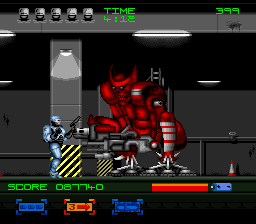In the image, a vibrant scene from a Robocop video game is depicted. Dominating the center is a towering red demon-like robot, resembling a crouching or sitting predator with hind legs similar to those of a frog. Its feet feature three prongs that provide stability, and as the legs ascend, they transition from red to silver with bold red stripes. The robot's upper body is entirely red, with a menacing face characterized by beady white eyes, red teeth, and horns, enhancing its demonic appearance. Large machine guns are mounted on its arms, emphasizing its threat. To the left of this intimidating figure stands Robocop, donning silver armor contrasted by black hands and a distinctive visor helmet that reveals only his mouth. In the top-left corner, five small Robocop icons represent lives, while green text indicates the time as 4:12 and the score as either 399 or 067740. A red health bar appears on the right side of the screen, positioned above additional icons—two blue, one orange, and a text indicating a count of three. The backdrop is an industrial hallway rendered in black and gray tones, adding to the game’s suspenseful atmosphere.